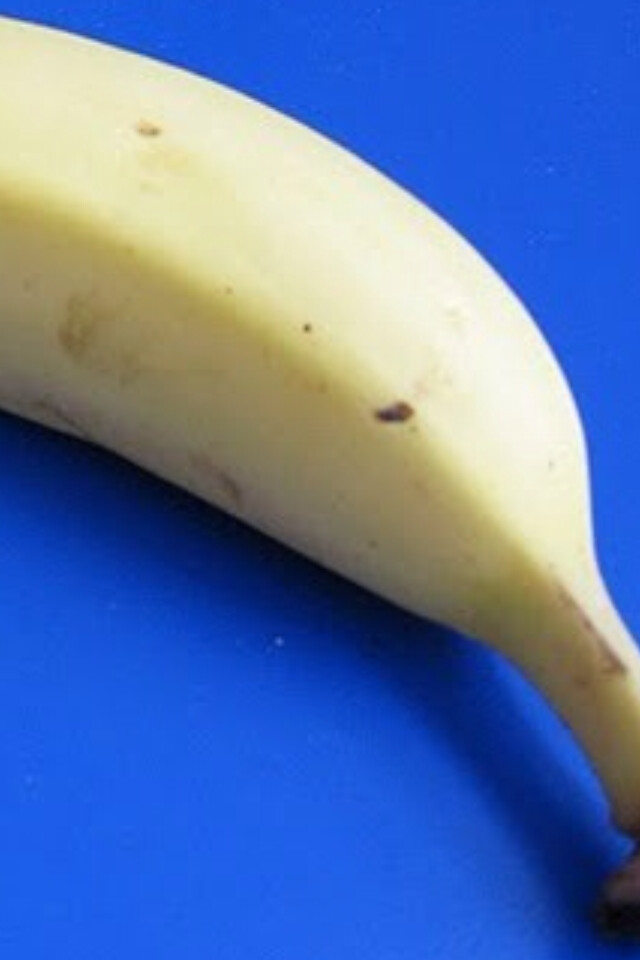An up-close image features a giant portion of a banana, occupying about a third to half of the frame. The background is a solid blue, though it’s unclear if the banana is on a counter, paper, or another surface. The banana itself is predominantly yellow, exhibiting only a few tiny brown specks and a slightly darker yellow area at the corner. The peel is a pale yellow hue with minor brown marks, approximately three on the lower part. The stem is mostly visible and remains closed, indicating the banana is unpeeled. Despite its imperfections, the banana appears fresh and ripe.